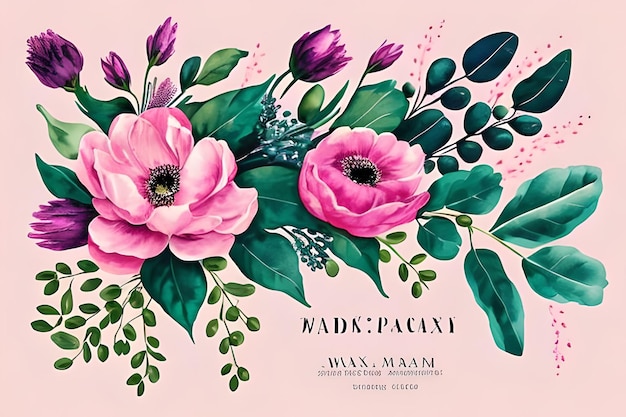This is an illustration, possibly digital, depicting a vibrant floral arrangement set against a light pink background. Dominating the center are two large pink flowers with black centers, surrounded by an array of green leaves in varying shades and watercolor-like textures. Interspersed among the foliage are smaller purple flowers, some of which appear to be tulips or berry-like buds. Tiny pink flowers, resembling dots, add delicate accents throughout the composition. At the bottom of the image is a block of text in black, difficult to read, but possibly containing names or event-related information in a non-English language, sprawled across several lines in a unique font. The image emits the feel of an invitation or poster, artfully balancing bold colors with intricate details.